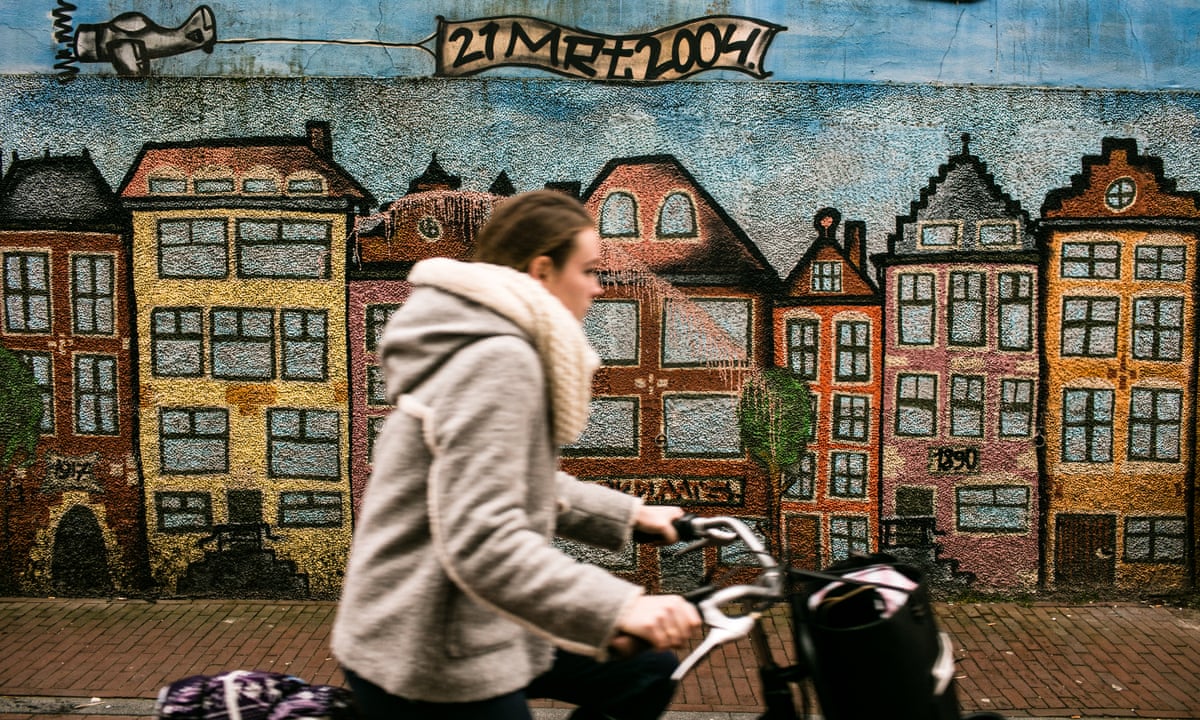The image captures a woman riding a bicycle from the left to the right side of the frame. She is in the foreground, wearing a gray hoodie with a white scarf, brown pants, and has brown hair. The bicycle features a black bag attached to the front. The photograph is slightly blurry, and the bike is visible only up to the handlebars before the image gets cut off around her waist. 

In the background, there's a mural painted on an old, dilapidated concrete wall. The mural depicts a vibrant cityscape with various colorful buildings that resemble European townhouses. These buildings are narrow and multi-story, painted in hues of brown, yellow, pink, and orange, set against a blue sky. Above the buildings in the mural, a cartoonish airplane is seen pulling a banner with the text "21 MRT 2004." Between the woman and the mural, a brick sidewalk is visible, adding depth to the scene.